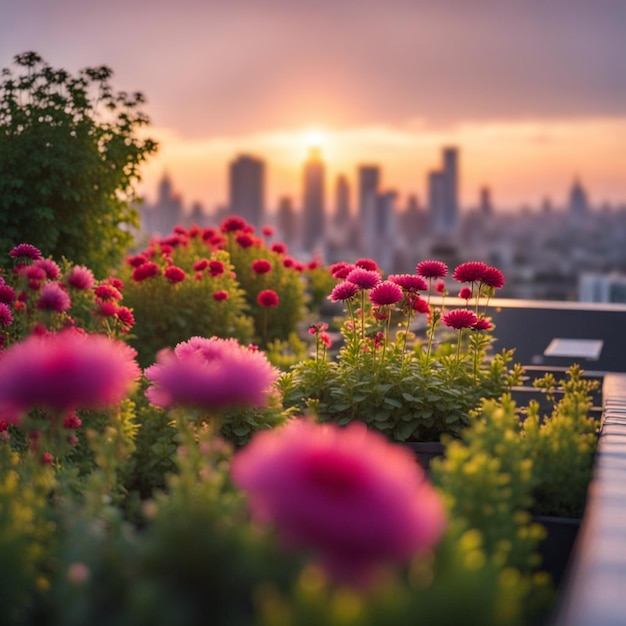This professional close-up shot captures a small urban garden perched atop a high-rise building, presenting an elegant contrast between nature and the cityscape. In the foreground, a lush assortment of vibrant purple flowers gracefully blends with rich green foliage, their details softened by a deliberate blur. As one's gaze moves deeper into the image, the flowers become sharply in focus, showcasing their beauty and intricate details. Encasing this rooftop oasis is a brick-lined planter, adding a rustic charm to the modern setting. Beyond the garden, the skyline of a bustling city—reminiscent of New York—is visible, rendered softly out of focus with tall skyscrapers silhouetted against a dramatic sky. The sky itself is a moody tableau, with dark gray clouds framing a setting sun that casts a golden-orange glow over the scene. This interplay of natural and man-made elements is further illuminated by the sun's soft, ethereal light, highlighting the tranquil beauty of the flowering plants against the dynamic backdrop of the city.